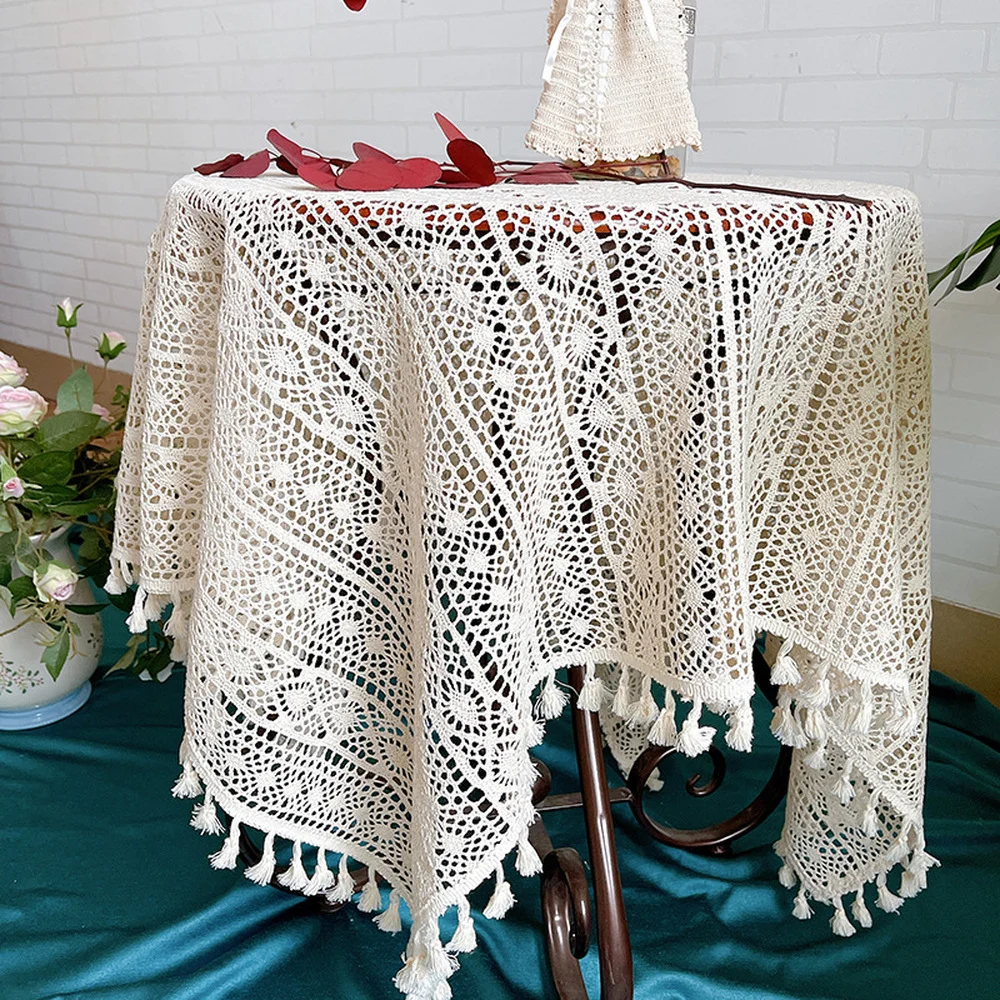The image captures a cozy room featuring a small round side table adorned with a delicate, see-through, crocheted white tablecloth that drapes gracefully over its surface. Although most of the table is obscured, the visible parts of the two brown legs spiral elegantly at their bases. On top of the table lies a long, stemmed branch adorned with striking red leaves, contributing a vibrant touch to the scene.

To the left of the table stands a decorative white pot embellished with a floral design, housing a thriving plant with lovely white and pink flowers. A second plant, positioned to the right of the table, adds to the room's botanical charm. The table and its decorations rest upon a draped aquamarine or teal material that covers the floor, enhancing the room's serene ambiance. The background features an aesthetically contrasting white stone wall, completing the picturesque setting.